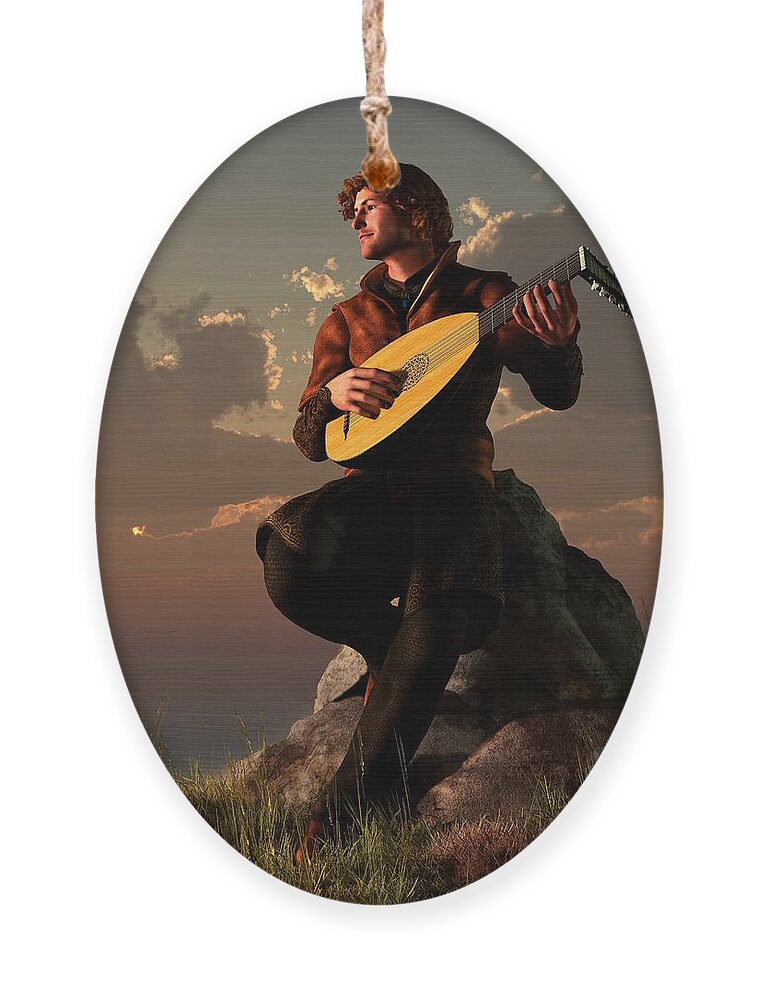The oval-shaped image is a photorealistic depiction of a young man with light, curly brown hair, playing a medieval-style stringed instrument resembling a lute. He is sitting on a rock amidst wispy grass, facing slightly to the left, and looks happy. He is wearing a quarter-zip, fall-orange jacket with darker sleeves and darker pants. The background features a moody sky, transitioning from a darker grayish-blue with dark gray clouds to peaks of pink and orange, suggestive of sunset. Despite a mysterious string hanging down above his head, partially covering the tip, his face remains clearly visible. The image focuses on his torso, face, and the instrument, with other details appearing softer in focus.